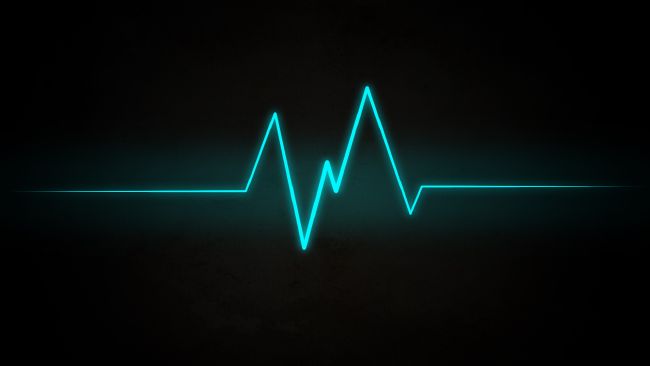The image depicts a graphic that closely resembles an EKG or heart monitor reading, set against a completely black background. Centered both vertically and horizontally within a horizontal rectangular frame, a neon blue line stands out vividly due to its bold color and slight neon glow. The line, which fades out towards the edges, alternates between peaks and valleys, capturing an irregular pattern typical of a heart monitor signal. Specifically, it features three upward peaks, one significant downward peak followed by a smaller downward peak, before leveling out twice along the horizontal axis. The simplicity and stark contrast of the bright neon blue against the pitch-black background create a visually striking and clean design.